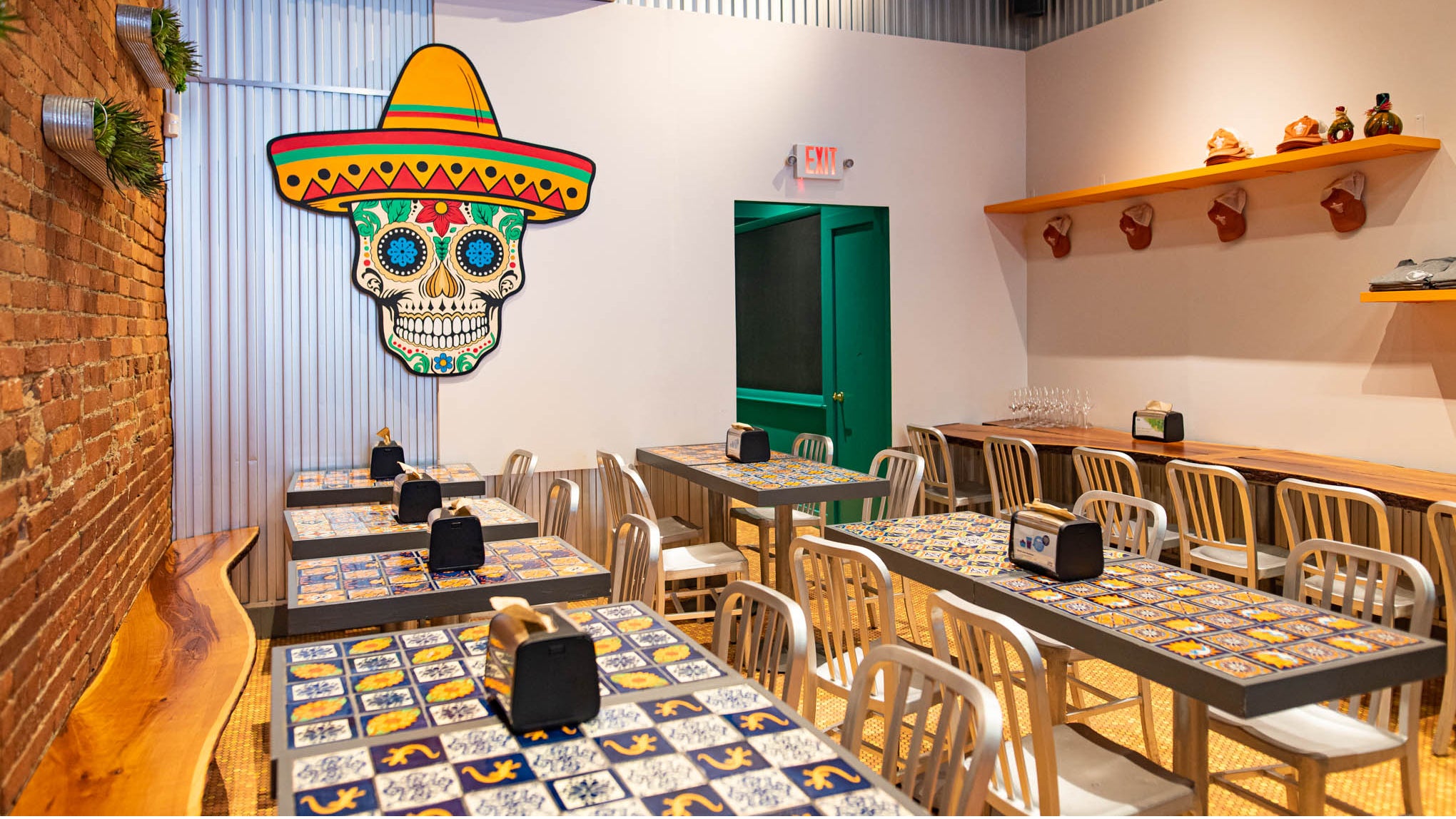The photo captures a vibrant dining hall of a Mexican or Spanish-themed restaurant. On the left side, there's a rustic brick wall adorned with a live wood-edged bench that appears to be made from the midsection of a tree. This bench is complemented by four tables showcasing intricate black, yellow, and white mosaic-like patterns, and silver-colored chairs positioned on the opposite side.

Hanging prominently in the room is a colorful "Day of the Dead" candy skull, adorned with floral patterns in green and red, and featuring bright, vibrant blue eyes. The skull wears a vivid sombrero with orange, green, and red patterns. The right side of the room houses additional tables with matching mosaic designs and an equal number of chairs on both sides. Further along the wall, there's another live wood-edged bench and a tabletop with chairs, alongside shelves that potentially display hats for sale.

The farthest corner of the room features a green exit way, adding a pop of color to the dynamic and culturally rich setting. The attention to detail, from the patterned tables to the decorative elements, creates an inviting and thematic dining experience.